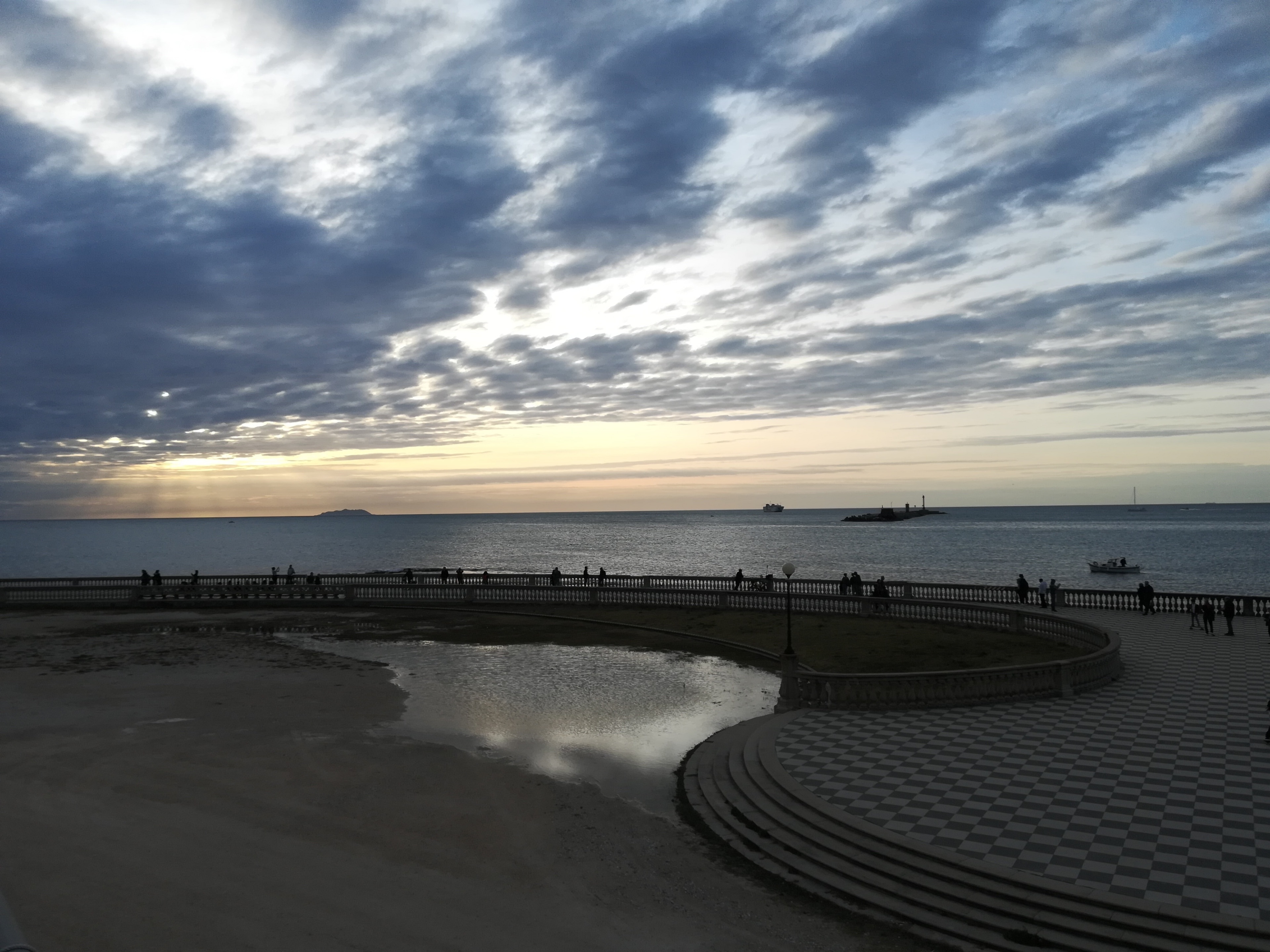This photograph captures a tranquil dusk scene by the coastline of a large body of water, likely the ocean or a sizable lake. The sky at the horizon is painted in faint hues of yellow and pink, transitioning to dark gray clouds above, suggesting an impending night. The calm water below mirrors the sky's muted palette, enhancing the serene atmosphere of the scene. A stone walkway and bridge stretch across the water, accompanied by a sandy area in the foreground. On this walkway, roughly two dozen indistinct figures stand, silhouetted against the fading light as they gaze out over the water. A non-illuminated street lamp along the railing adds a charming, yet somber touch. In the distance, a large, nearly indistinguishable ship looms, while a smaller boat is situated closer to the foreground. The overall color scheme—dominated by shades of blue, black, and gray—adds to the twilight ambiance, making for a picturesque and reflective moment.